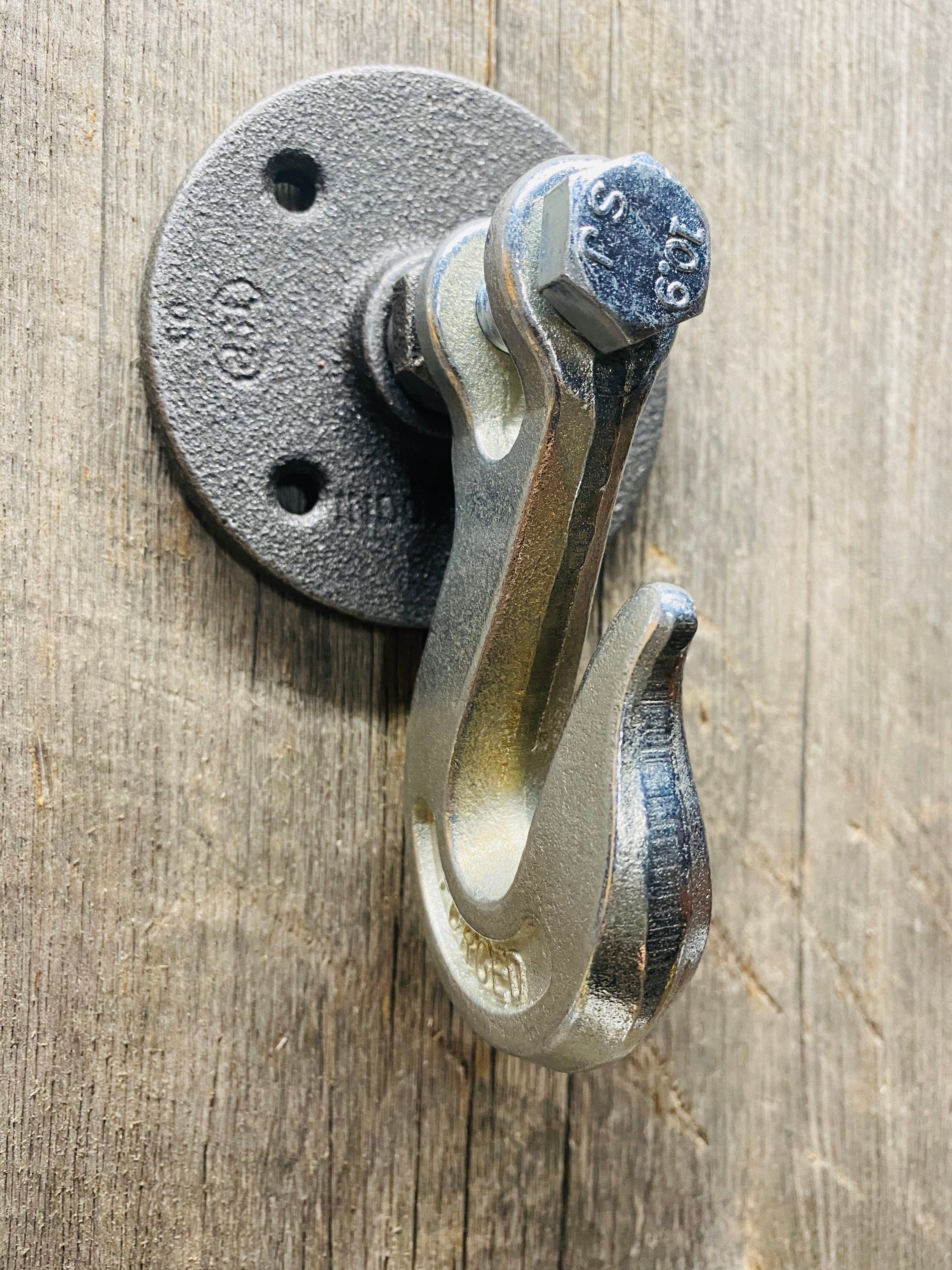The image is a high-definition close-up of a heavy-duty hook mounted on an old, worn, light brown wooden wall or door. The wooden surface features visible scratches, particularly to the right of the hook. The hook itself is large and thick, made of shiny silver metal, and curves in a half-S or J shape. It protrudes from a black circular mounting plate affixed to the wood, which has several holes with screws or bolts securing it. At the top of the hook, there is a hexagon-shaped bolt engraved with the letters and numbers "RS 10.9 SJ." The bolt is oriented so its text reads properly when viewed from the left. The hook also has some additional, less discernible writing imprinted onto it. Overall, the detailed combination of these elements suggests a robust and well-secured hanging mechanism.